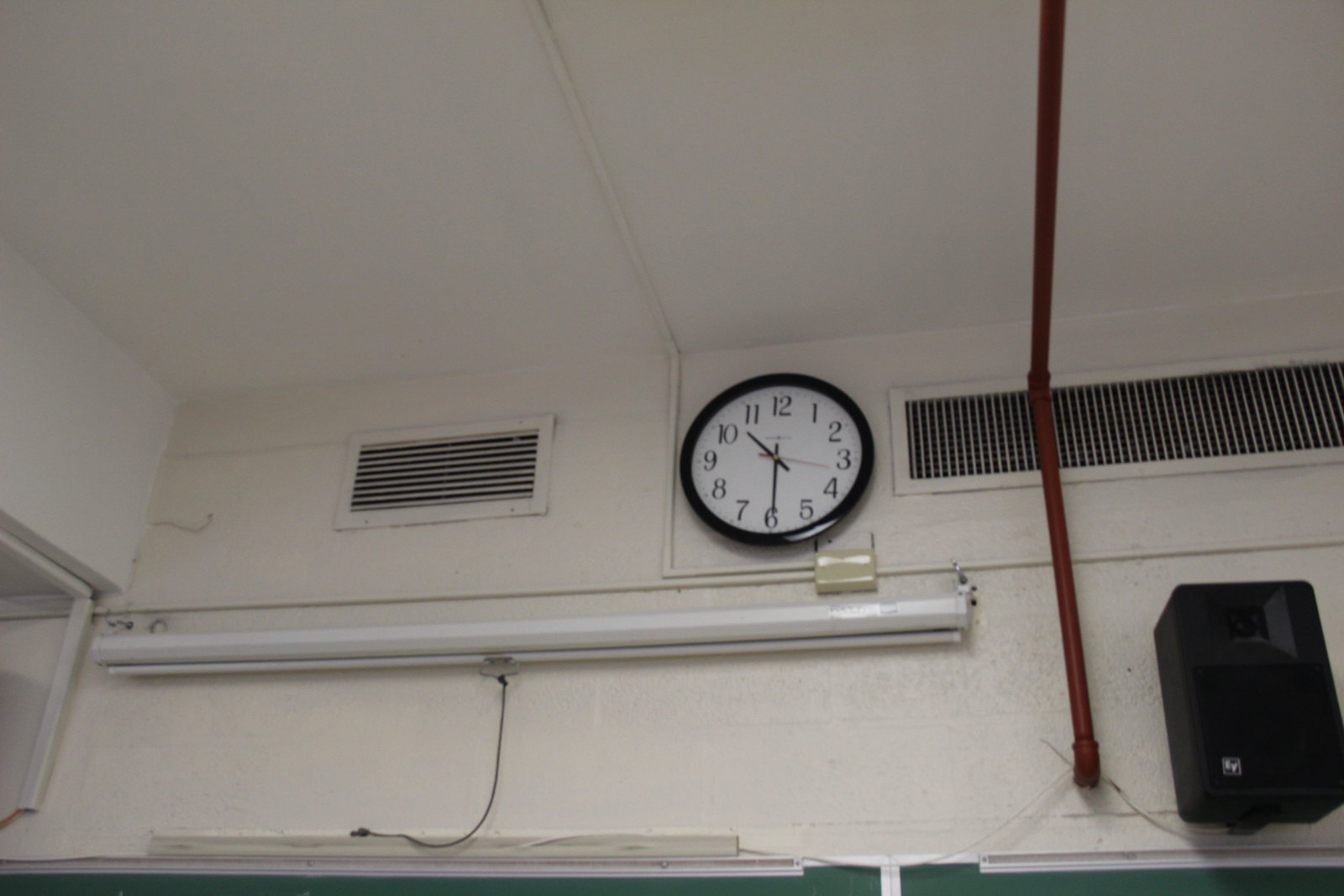This photograph captures the upper section of a classroom wall, evoking a sense of old school settings. Dominating the center is an analog clock with a black frame, a white face, black numerals, and black hash marks. The clock's hour hand points between 10 and 11, the minute hand rests at the 6, and the red second hand is a quarter past the 3, indicating 10:30. To the right of the clock, a maroon-colored pipe juts out horizontally from the white wall, intersecting a large rectangular white vent. On the left, there is a smaller, white rectangular vent. Below the clock, a white rolled-up projector screen with a black cord drapes down, ready to be pulled for use during class. Additionally, the edges of dark green chalkboards with silver borders frame the lower part of the wall. A black rectangular speaker is also mounted on the wall. The entire setting is bathed in light from the stark white walls and ceiling.